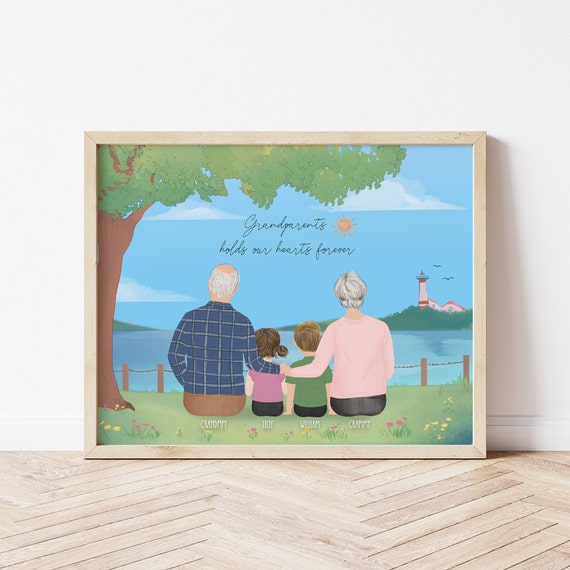This is a detailed image framed in light-colored wood, almost matching the light brown, zigzag-patterned floor it leans against. The background features an off-white or white wall. The frame encloses an evocative painting or colorful photo of four individuals—a pair of grandparents on either side and their two grandchildren in the middle. The grandparents, with gray hair, are embracing the children: a girl with her black hair in double ponytails and a boy with short-cropped brown hair. They sit on a grassy landscape, their backs to the viewer, gazing out over a serene body of water. Above them, a tree with a lush green canopy extends over the left side of the image. The water stretches toward a distant, greenery-filled land where a white lighthouse with red stripes stands, accompanied by two smaller buildings and a spit of land visible to the left. The blue sky above is dotted with three clouds and two seagulls in silhouette. The picture features the heartfelt text "Grandparents hold our hearts forever" in black letters at its center, encapsulating the familial bond portrayed. A small, unobtrusive metal fence or line and some wood poles are visible near the water's edge, perhaps for safety.